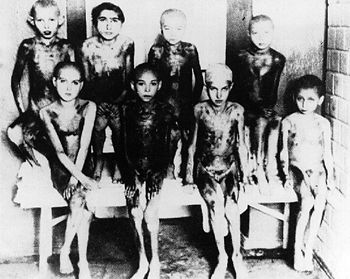The black and white photograph, possibly taken in the 1940s or 1950s, is a haunting image of eight emaciated children, both boys and girls, seated in two rows against a stark block or brick wall. The rectangular, almost square image captures the children in a disturbing, malnourished state with visible ribs and bone structure, suggesting severe famine or the aftermath of a chemical spill. They appear either nude or scantily covered, further adding to the distressing nature of the scene. The children have somber, haunted expressions as they stare directly at the camera, their thin limbs and bruised bodies starkly highlighted in the monochrome palette. The setting includes a bench or table-like structure upon which they sit, enhancing the image's historical and melancholic aura.